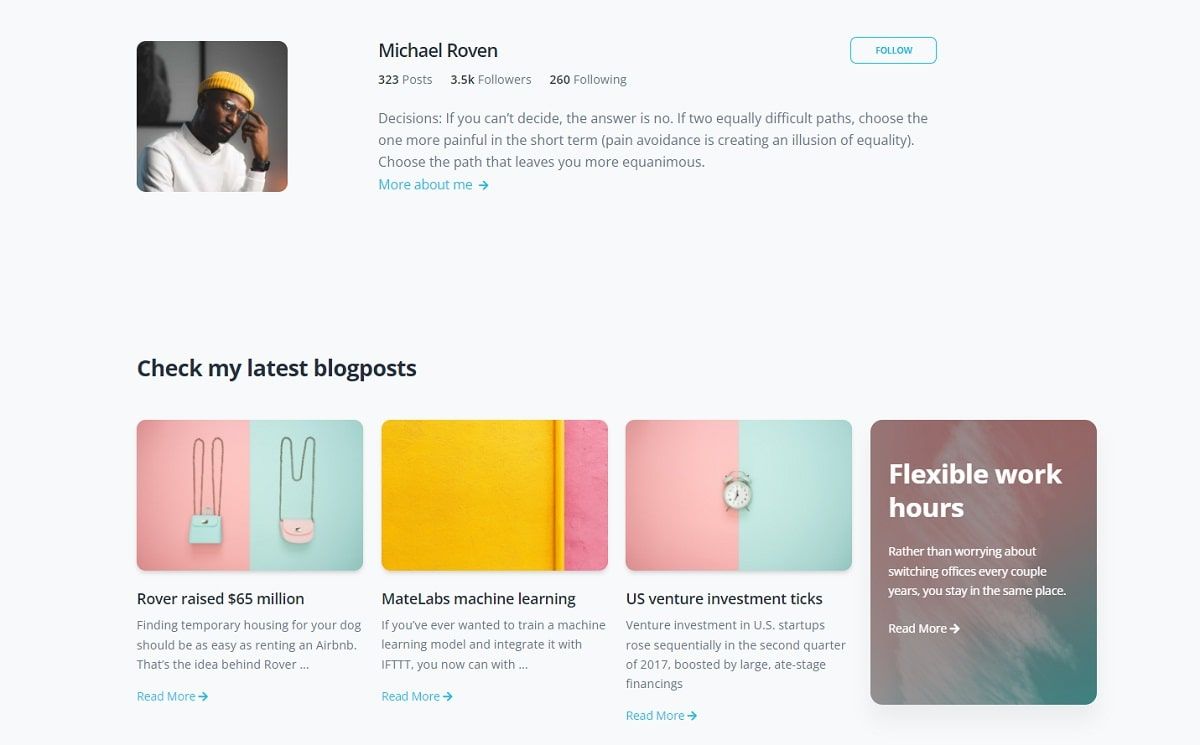This image, sourced from a website, showcases a profile section prominently displayed at the top left. The profile features a man named Michael Rovin, who is wearing a distinctive yellow hat. Adjacent to his photo is a summary of his social media activity, including "323 posts," "3.5k followers," and "260 following," along with a "Follow" button. Below his stats, there's a motivational description detailing his philosophy on decision-making: "If you can't decide, the answer is no. If two equally difficult paths, choose the one more painful in the short term. Pain avoidance is creating an illusion of equality. Choose the path that leaves you more equanimous." Directly beneath this description, there's a call to action urging visitors to "Check my latest blog post."

The image also features a section with blog post titles: one notable post titled "Rover Raises $68 Million," another on "PostMate Labs Machine Learning," and a third discussing "U.S. Venture Investment Tricks."

In the bottom right corner, there's a grayish box with white text that reads: "Flexible work hours—rather than worrying about switching offices every couple of years, stay in the same place. Read more," accompanied by an arrow pointing to the right.